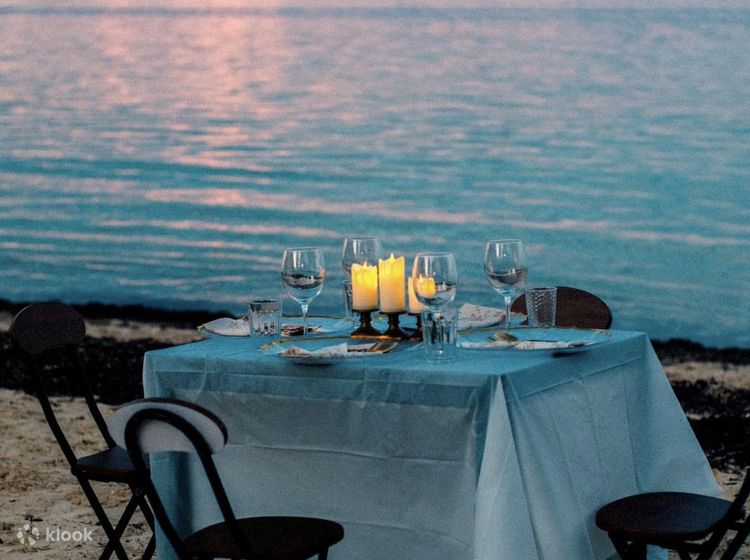This photograph captures an elegantly set dining table positioned directly on the sandy beach, in close proximity to a serene, expansive ocean. The table, draped with a blue tablecloth that flutters gently in the breeze, is meticulously arranged with fine dining ware including four half-filled wine goblets, secondary glasses, clear plates, and an assortment of silverware. In the center of the table, three lit candles contribute to the intimate, celebratory atmosphere, perfect for a special occasion such as a wedding reception. Surrounding the table are four black folding chairs, neatly tucked in, suggesting readiness for an unforgettable seaside meal. The scene is bathed in the warm, pinkish hues of a setting sun, whose rays reflect softly upon the calm waters, enhancing the romantic and tranquil ambiance. Alongside the sandy shoreline, small clumps of seaweed are visible, underscoring the natural beach setting of this picturesque evening.